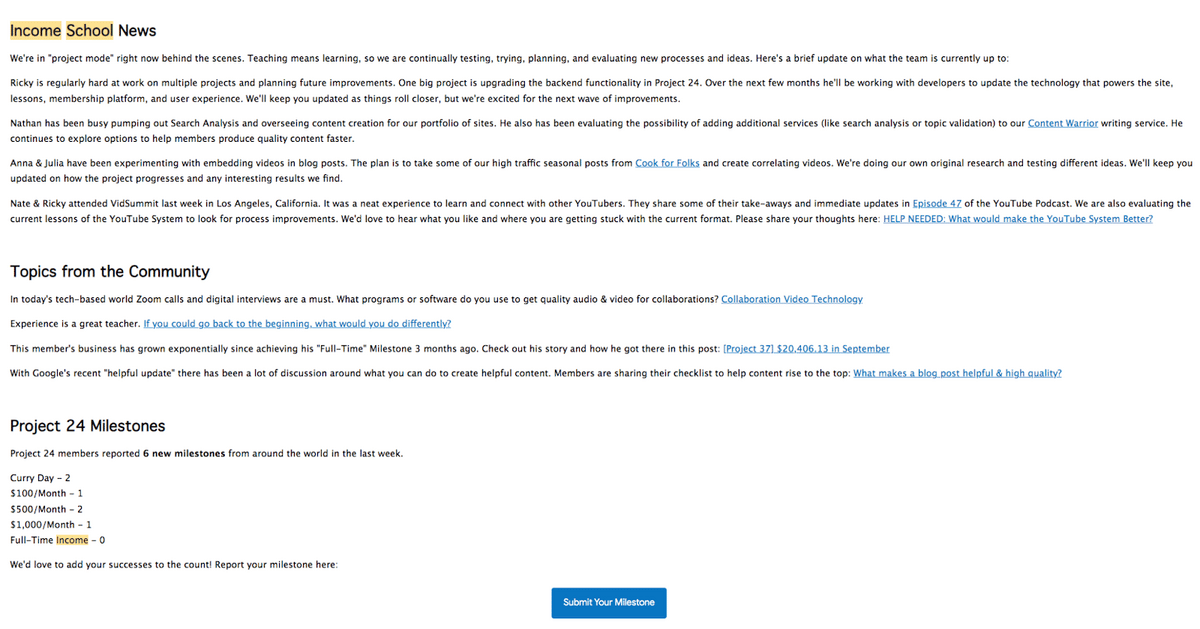### Income School News Update: Project Insights and Team Endeavors

**Current Status and Team Activities**

This image captures a comprehensive update from "Income School News". The team is currently in an intense project mode, focusing on learning through teaching, which entails continuous testing, planning, evaluating, and trying new strategies.

**Ricky's Multi-Project Management**

Ricky is diligently working on multiple fronts. A major initiative he is spearheading involves upgrading the backend functionality of Project 24. Over the next few months, Ricky will collaborate with developers to advance the technology that underpins the core components of Project 24, including the site’s infrastructure, lessons, membership platforms, and overall user experience. The team is enthusiastic about the forthcoming improvements and will keep everyone updated as developments unfold.

**Nathan's Search Analysis & Content Supervision**

Nathan is immersed in performing thorough search analyses and overseeing the content creation for a variety of sites within the team's portfolio. He is also evaluating the potential addition of new services to the Content Warrior Writing Service, such as search analysis or topic validation. His goal is to streamline the process to enable members to produce higher-quality content more efficiently.

**Anna and Julia’s Video Integration Experiment**

Anna and Julia are pioneering the integration of videos into blog posts, particularly focusing on high-traffic seasonal content from the "Cook for Folks" blog. They are conducting original research and experimenting with different approaches. Updates on the project's progress and any interesting findings will be shared in due course.

**VidSummit Insights**

Recently, Nate and Ricky attended VidSummit in Los Angeles, California. They found the experience valuable, with opportunities to connect with other YouTubers. Their insights and immediate takeaways can be found in episode 47 of the YouTube podcast. Additionally, the team is reviewing the current YouTube system lessons to identify potential process improvements and is soliciting feedback from the community to enhance the system further.

**Community Interaction and Feedback Requests**

- **YouTube System Improvements**: The team invites members to share their likes and challenges with the existing YouTube system.
- **Collaboration Tools**: Inquires about preferred programs or software used for high-quality audio and video in digital collaborations.
- **Learning from Experience**: Engages members to reflect on their journey and think about what they would have done differently from the start.

**Project 37 and Income Milestones**

There is also an insightful case study of "Project 37", revealing earnings of $20,406.13 in September. The discussion extends to strategies for creating helpful content, inspired by Google's recent update. Members are exchanging checklists for content improvement.

The team celebrates Project 24 milestones, announcing six new achievements from around the globe in the past week, and encourages others to report their successes.

**Call to Action**

At the bottom of the update, a prominent rectangle invites members to "Submit Your Milestone," encouraging the community to share their accomplishments and contribute to the collective progress.